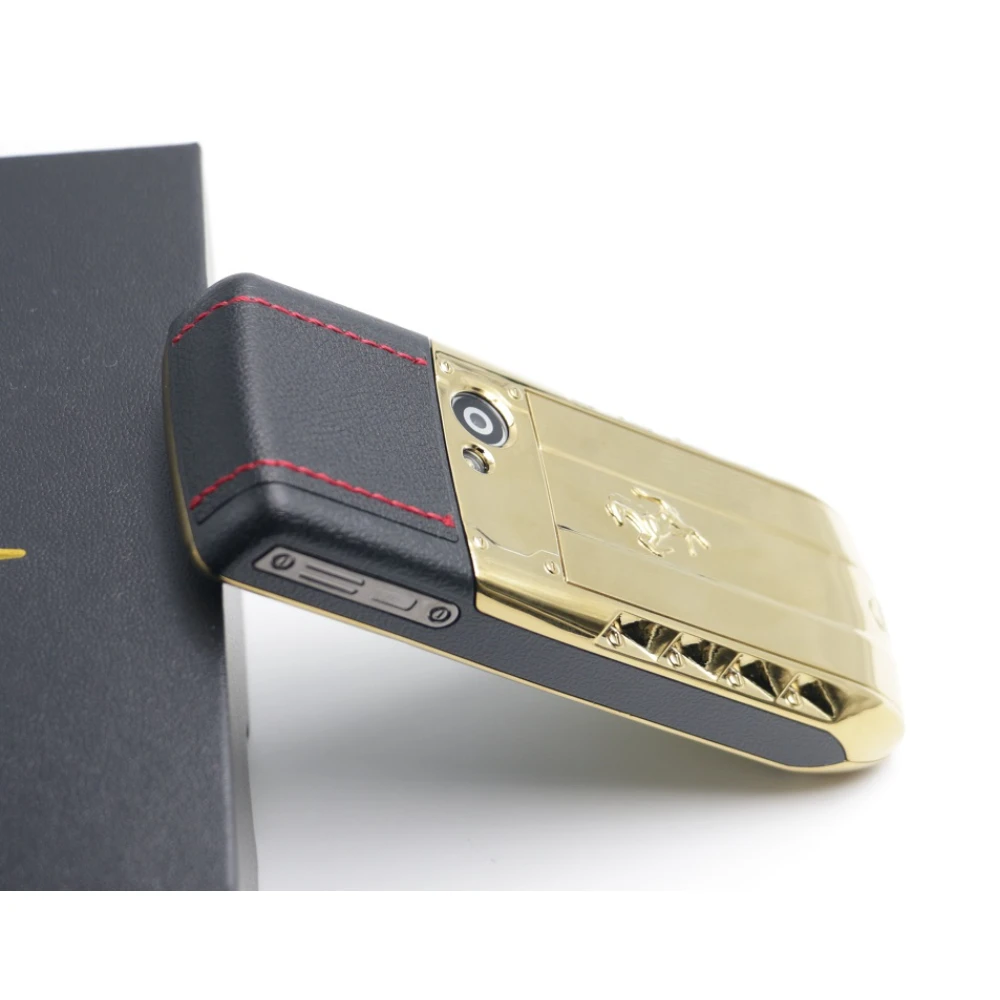The image features a sleek device, most likely an old phone or compact camera, adorned with a gold-plated back that showcases a prancing horse, reminiscent of the Ferrari logo. The device is encased in a black leather cover with intricate red stitching, featuring two parallel strips of red threading. Positioned on the right side, the device is slanted against a long, black rectangular object, potentially a decorative element or piece of wood. Surrounding the camera lens on the gold plating, there are several holes or ports, possibly for charging or other electronic functions. The left side of the image includes a possible graphite-colored gift box, set against a white background. Silver detailing with three buttons is observed along the side of the device, enhancing its sophisticated design.